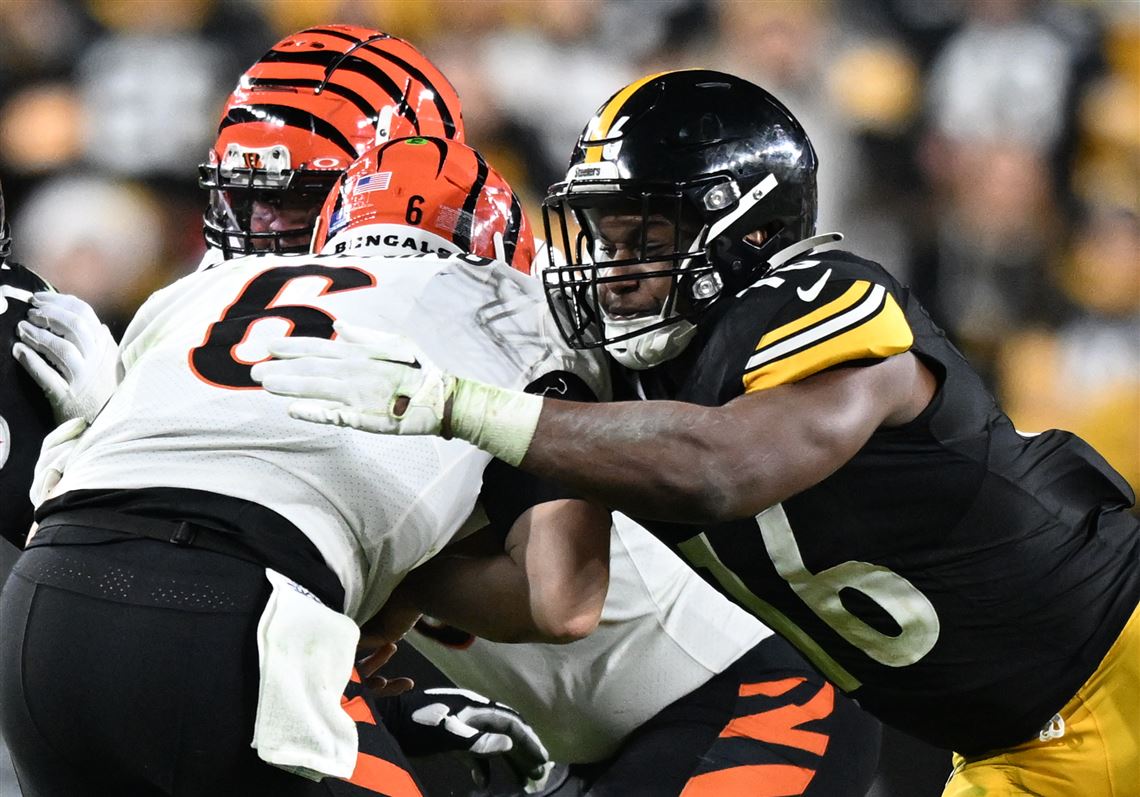In this dynamic action shot from an NFL game, we see players from the Cincinnati Bengals and the Pittsburgh Steelers engaged in an intense play. At the center of the scene, Bengals player number 6, wearing a white jersey with black pants featuring black and orange stripes, is leaning forward, seemingly clutching the football. His helmet is distinct with black and orange tiger stripes, and it reads "Bengals" across the bottom. Behind him, reaching out in an attempt to tackle, is Steelers player number 16. He is clad in a black jersey with white lettering, yellow pants, and a black helmet with a yellow stripe down the middle. Number 16's gloved hand is firmly on number 6’s back. The background is artistically blurred with a bokeh effect, revealing a sea of indistinct spectators in the stands, their colors merging into splotches of white, yellow, and black. This image captures the essence of the competitive clash between the two teams, highlighting their iconic uniforms and the high-stakes action on the field.